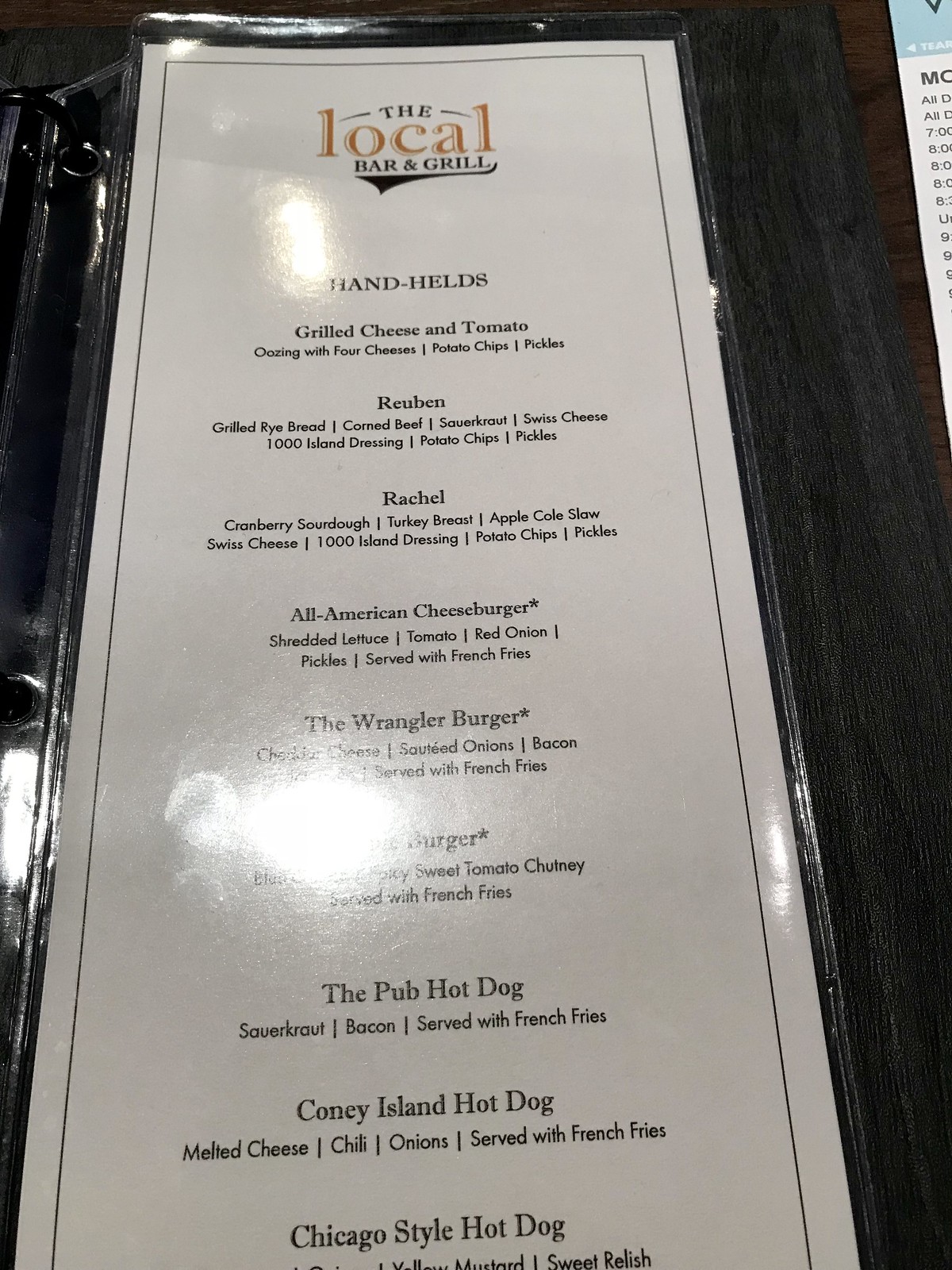This is a detailed color photograph in portrait orientation capturing a menu encased in clear plastic. The menu features a clean, white background with the heading "The Local Bar and Grill" prominently displayed at the top. The word "Local" is elegantly rendered in gold, while the rest of the text is in black. Intrusively, the upper right corner of the image shows a glimpse of another menu, though it’s difficult to discern beyond some visible text.

The menu lists a variety of handheld options, including sandwiches, burgers, and hot dogs. Specific offerings include:

- Grilled Cheese and Tomato
- Reuben
- Rachel
- All-American Cheeseburger
- The Wrangler Burger
- The Burger
- Pub Hot Dog
- Coney Island Hot Dog
- Chicago-style Hot Dog

Each item is accompanied by a brief, yet informative description. Noticeably, the menu does not provide prices for these items. The burgers and hot dogs are served with French fries, while the sandwiches come with potato chips and pickles.